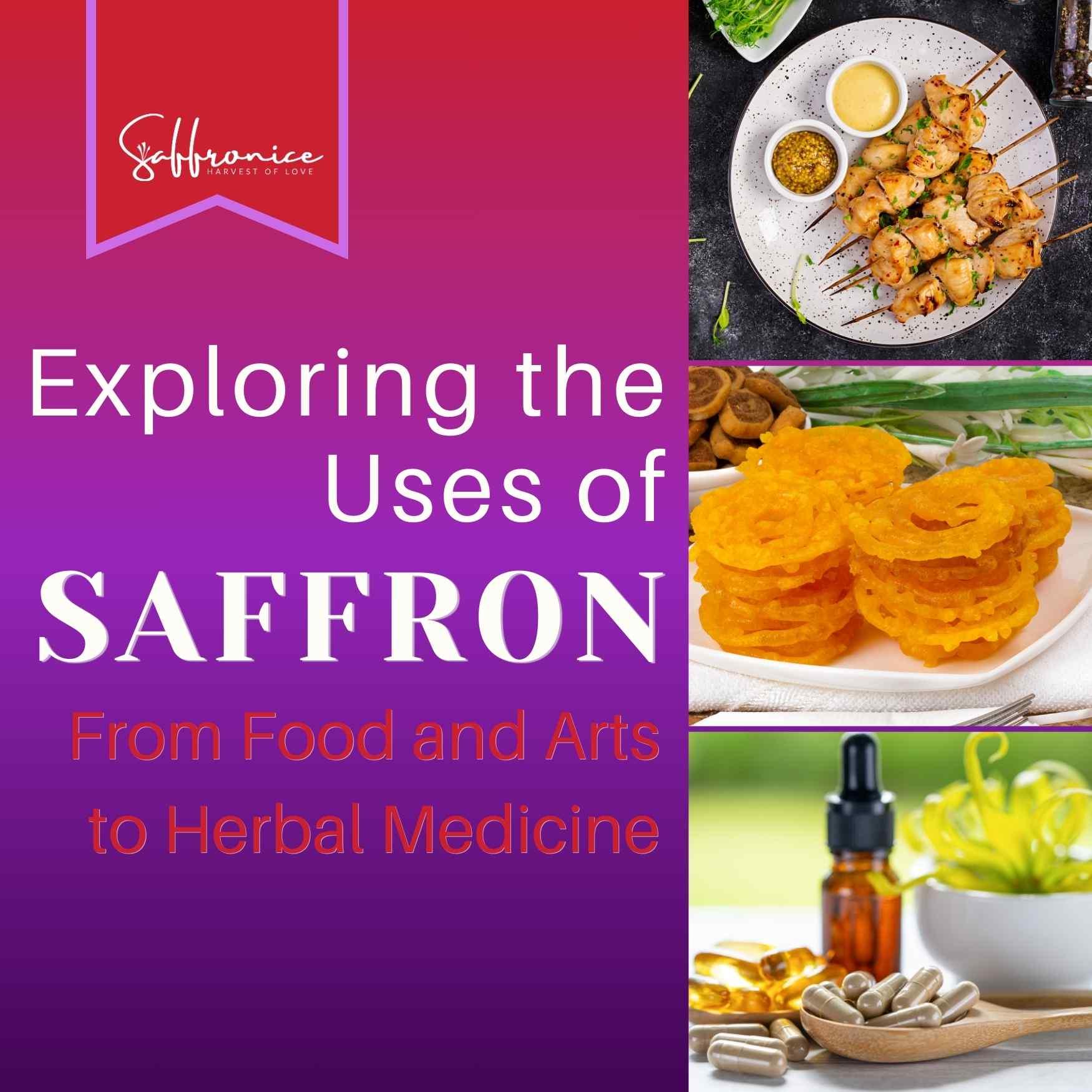The infographic, presented by the company Saffronice, Harvest of Love, is titled "Exploring the Uses of Saffron from Food and Arts to Herbal Medicine." The background transitions from radiant pink at the top to deep purple at the bottom, with the title prominently displayed at the top left. The right section of the image features three photos aligned vertically. The first photo showcases a white plate with skewered kebabs, adorned with potential saffron sprinkles and accompanied by two dipping sauces—one yellowish and buttery, the other thick and chunky, possibly resembling baba ghanoush, with additional green herbs seen in the background. The second photo displays a stack of onion-ring-like items on a white plate, with what appear to be cinnamon buns and more green herbs in the background. The third photo illustrates a brown eyedropper bottle with a black cap, two wooden spoons with tan and yellowish caplets, some tan caplets scattered on the counter, and a white bowl with green herbs in the background.